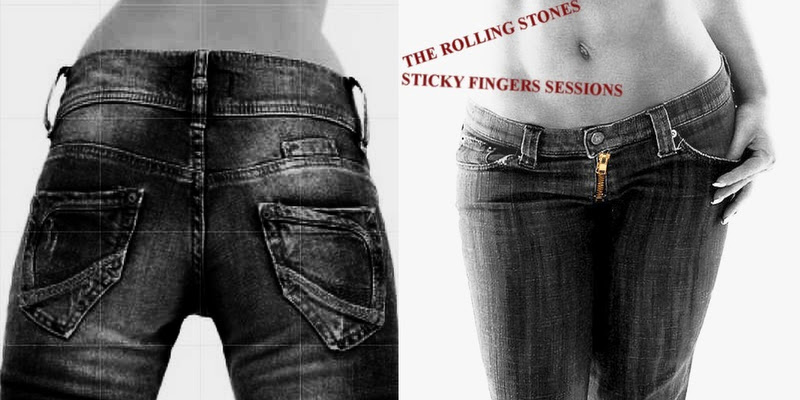This black and white media piece consists of two side-by-side photographs associated with the Rolling Stones' Sticky Fingers sessions. The left image captures the back view of a woman in blue jeans, distinctly showing the pockets with pointed bottoms and a sliver of her bare back, indicating she is not wearing a shirt. The right image presents the same woman from the front, highlighting her flat midriff and well-manicured white nails. Her left hand rests on her hip with the thumb slightly tucked into her pocket. Notably, the zipper on the jeans is tinted a striking bright brass color and stands out in the monochromatic setting. Spanning both images in a dark red, Times New Roman-like font are the words "The Rolling Stones Sticky Fingers Sessions."